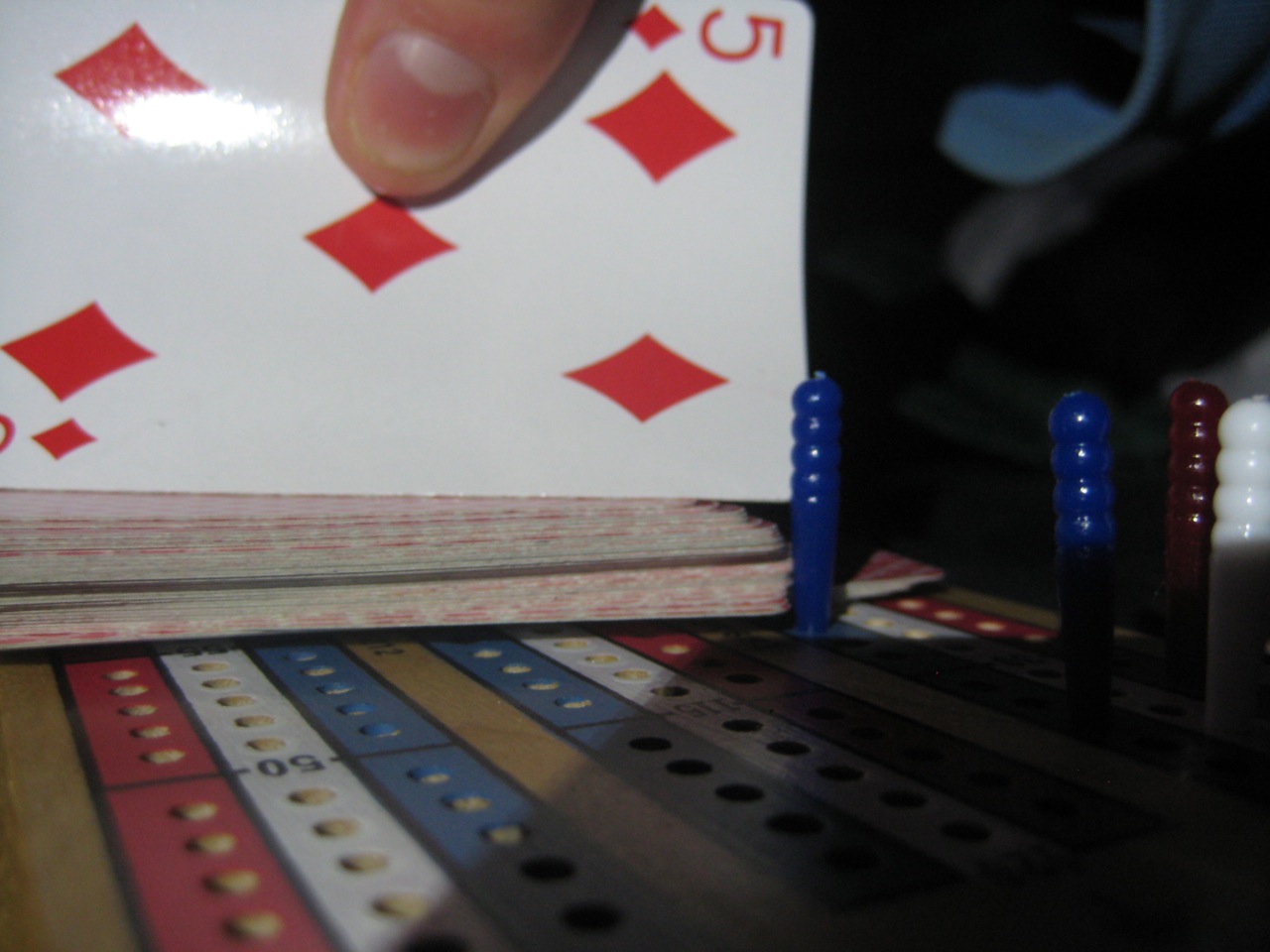In the photograph, a hand enters from the top left corner, with fingers holding a playing card upright on its edge. The card is the five of diamonds, featuring a '5' in both top corners, each accompanied by a small diamond icon beneath it. The card itself displays five diamond symbols in a standard arrangement, and a slight glare reflects off its surface. Below the suspended card, a deck of cards is neatly stacked. Further down, there is a game board with multiple rows of colored holes. Specifically, there are two blue pegs, one red peg, and one white peg placed within these rows. The rows are organized by color—red, white, and blue—each with a series of holes and the number '50' marked on the initial rows. The pattern of red, white, and blue rows repeats across different sections of the board, each section lined with holes corresponding to their peg colors.